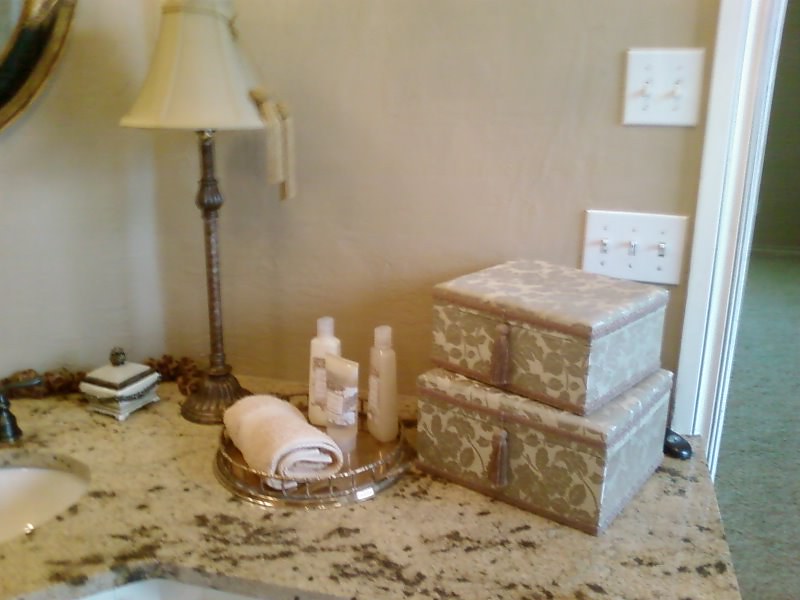The image captures a meticulously arranged bathroom counter corner. On the left, a white sink basin is seamlessly incorporated into the beige, marbleized countertop, paired with a sleek black faucet. A tall, slender copper lamp with a beige lampshade adorned with two hanging tassels stands on the counter, casting a warm glow. Next to the lamp, a petite black and white ceramic square dish rests elegantly. 

To the right, a sophisticated vanity organizer, an elegant blend of silver and shiny gold with a mirrored base, houses a neatly rolled beige towel. Accompanying the towel are two bottles, likely containing hand soap or shampoo and conditioner, and a centrally placed squeezable lotion bottle.

On the far right of the countertop, two identical decorative boxes, the smaller perched atop the larger, feature beige and olive green leaf patterns and are accentuated by matching tassels. The bathroom wall and door frame are painted beige, with the door itself in a crisp white. 

Adjacent to the doorway, a pair of light switches share a socket at the top of the wall, while about a foot below, three more switches are aligned, all in the on position, ensuring an illuminated and welcoming atmosphere.